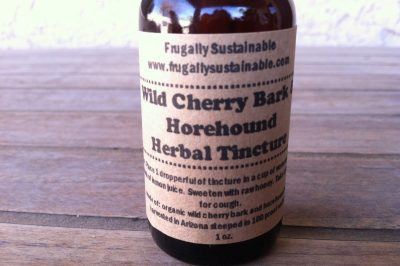The photograph features an amber-colored glass bottle positioned on a wooden table with a clear wood grain pattern. The image primarily focuses on the label of this partially visible bottle, which has a handcrafted, beige, kraft paper look. The label has large, black printed text and reads: "Frugally Sustainable" with the website "www.frugallysustainable.com" followed by a series of dots. Below this, in larger type, it states "Wild Cherry Bark, Whorehound, Herbal Tincture." Further text includes dosage instructions: "One dropper full of the tincture in a cup," and it mentions using lemon juice sweetened with raw honey as a remedy for coughs. Though partially out of focus, additional text suggests organic ingredients and notes that the bottle contains one ounce of the tincture. The photograph seems to have been taken outdoors, reflected by the blue sky and trees seen on the bottle's surface.